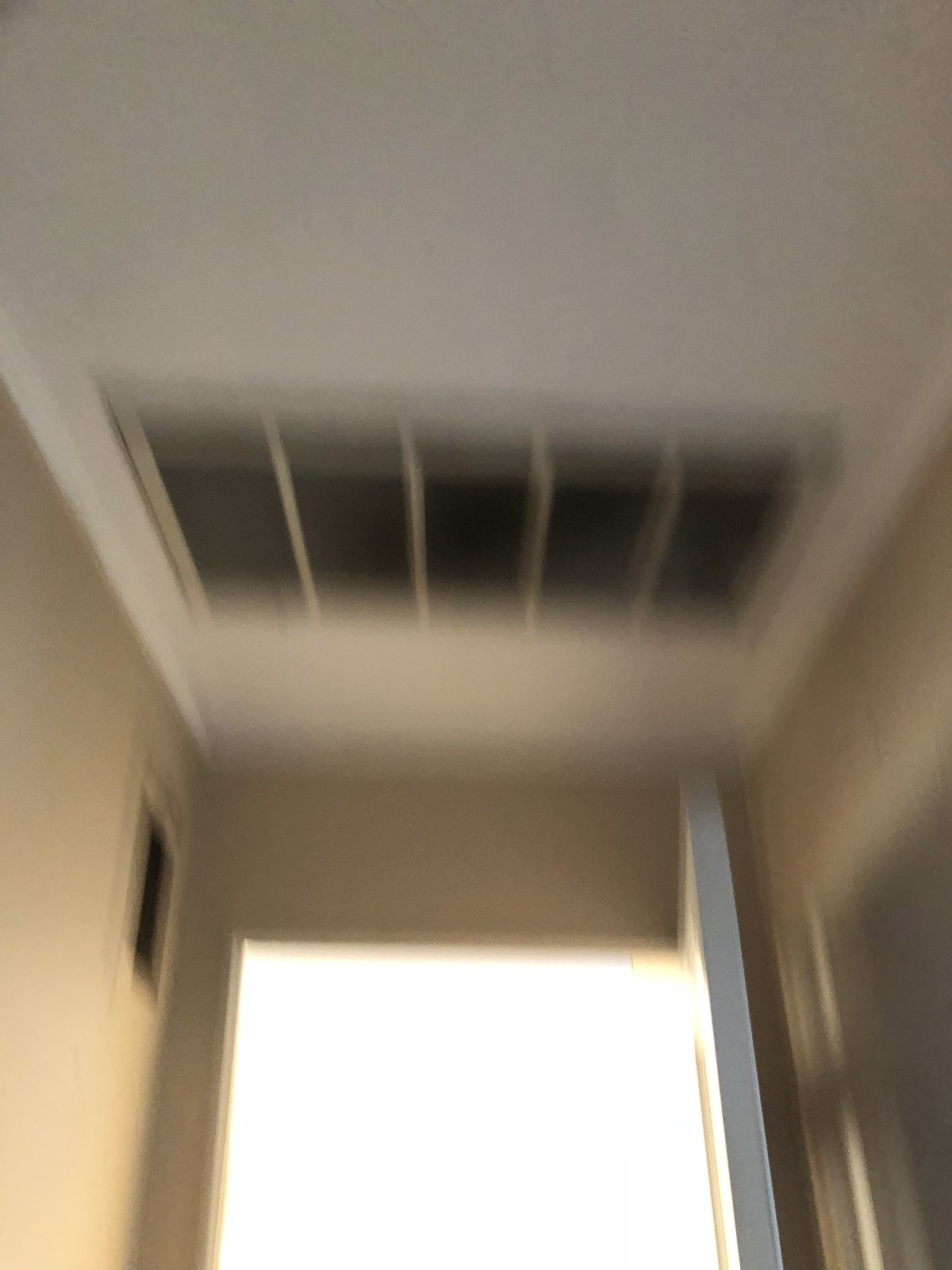A spacious hallway inside a house is depicted in the image. The hallway features beige walls and a pristine white ceiling from which a noticeably dirty ceiling vent hangs; black dust is visibly accumulated on it. Additionally, there is a smaller vent on the right side of the ceiling that is similarly encrusted with black dust. To the left, an open white door reveals a flood of bright, white light pouring into the hallway, creating stark shadows in its wake. However, the room beyond the door remains concealed. The open door's frame casts multiple shadows across the floor and walls, adding depth to the scene.